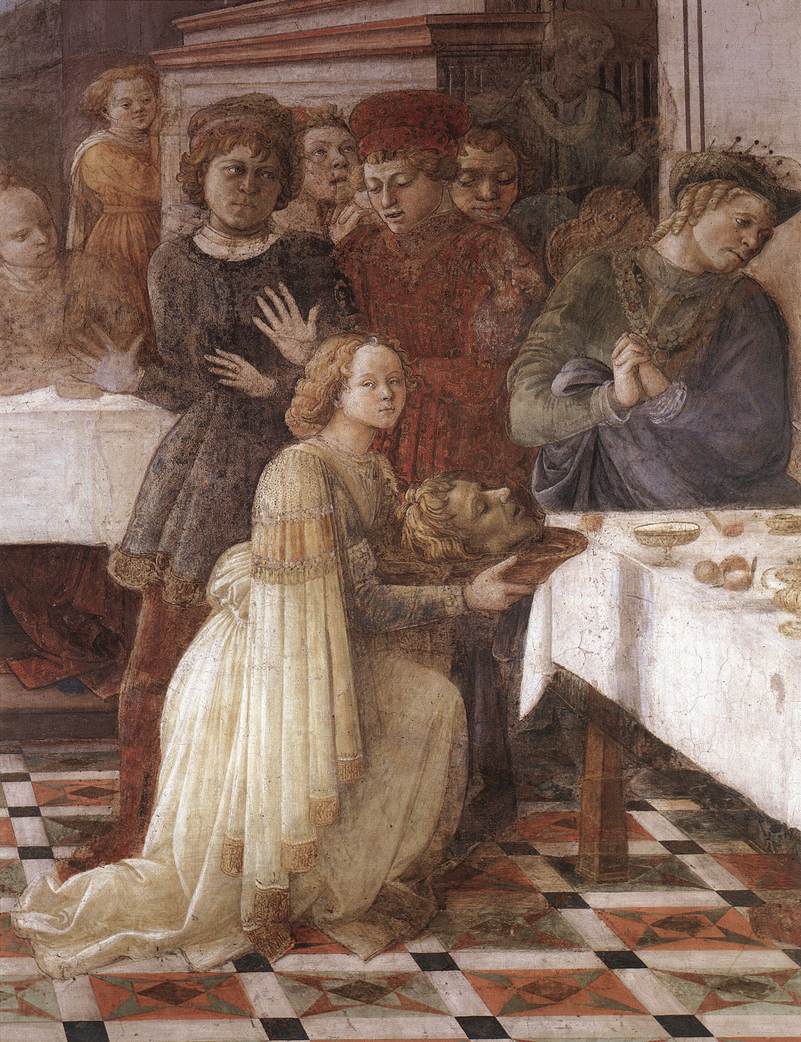The painting is a tall, rectangular artwork set in a grand dining room during a dramatic feast. The floor features intricate tile work with a pattern of crossing white and black squares adorned with triangular designs. On the left and right bottom corners are large tables draped in white tablecloths. The scene centers around a young woman in a long, drapey gown of beige and light orange, who is kneeling and presenting a platter with the severed head of a man, likely John the Baptist, to a master at the table. Her expression is somber and she looks directly towards us. Surrounding her are numerous figures, some appearing as youthful servants or squires, engaged in conversations or displaying emotions of anguish and concern. The background reveals additional figures and a ghostly presence watching over the scene, adding to the air of tension and unease. The people are dressed in renaissance-style clothing, and the overall atmosphere is one of an ornate yet grim banquet, with an event that has left the attendees visibly shaken.